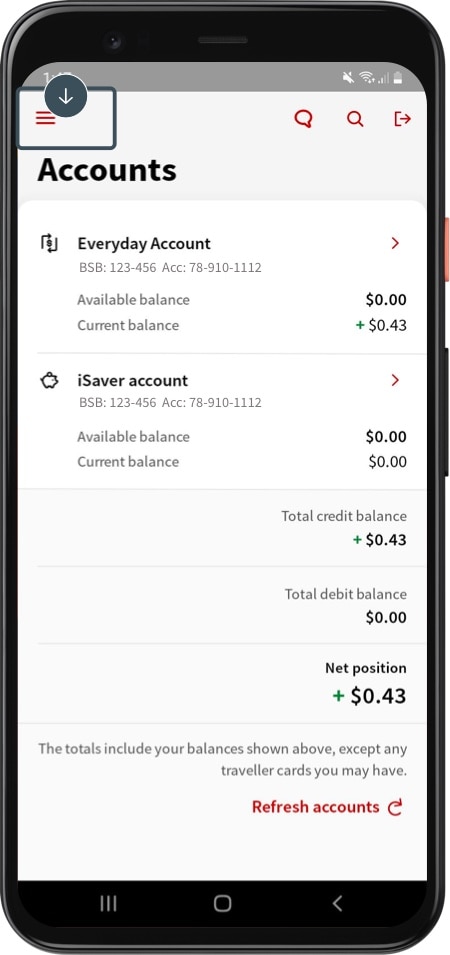This image features a smartphone with a noticeably edited screen display, resembling a tutorial interface. The smartphone has black bezels, and at the bottom of the screen, there is a navigation bar with home, back, and minimize buttons. The screen itself is primarily white with shades of gray at the top.

At the top of the screen, a light gray rectangle prominently displays the text "Accounts" in black font. In the upper right corner of this section, there are three icons: a speech bubble, a magnifying glass, and a back arrow.

Above the word "Accounts," three horizontally-aligned lines are displayed vertically, possibly indicating a menu. A gray rectangle with an arrow pointing at these lines suggests an instructional element. Below this indicator, another white rectangle bears the text "Everyday Account." 

The account details are meticulously displayed: 
- BSB: 123-456
- Account: 78-910-1112

It also shows financial information:
- Available balance: $0.00
- Current balance: +$0.43